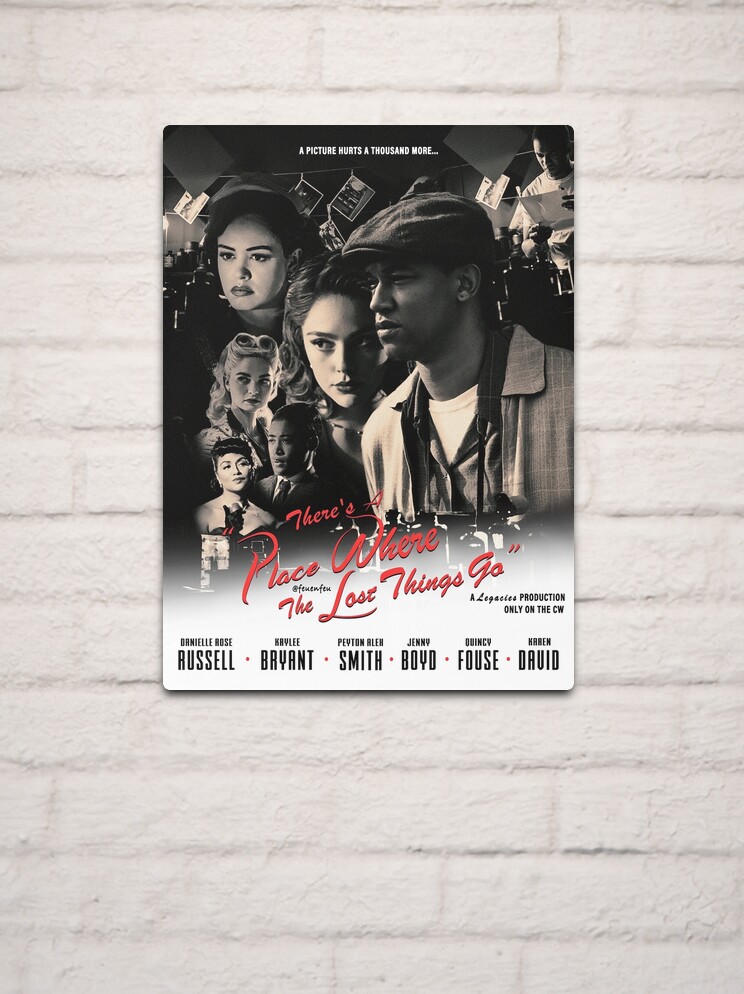The movie poster titled "There's a Place Where the Lost Things Go" is displayed against a realistic whitewashed brick wall, giving the image a blend of photographic and illustrative elements. Above the title, the tagline reads, “A picture hurts a thousand more.” This black-and-white poster features a diverse cast of six characters styled in 1950s attire. At the center-right, the main character, an African American man, is depicted wearing a beanie-style cap and a tweed jacket. To his left, three women are shown, adorned with fifties-style makeup, hair, and accessories. Below them, a man and a woman are similarly dressed in mid-20th-century clothing. Despite some illegible parts, the cast list includes names like Darryl Reyes-Russell, Kaylee Bryant, and likely Arnell Rose Bryant and Ginny Boyd, among others. The entire scene conveys a historical ambiance, possibly linking back to the 1920s or 1930s, and suggests a narrative steeped in the past.